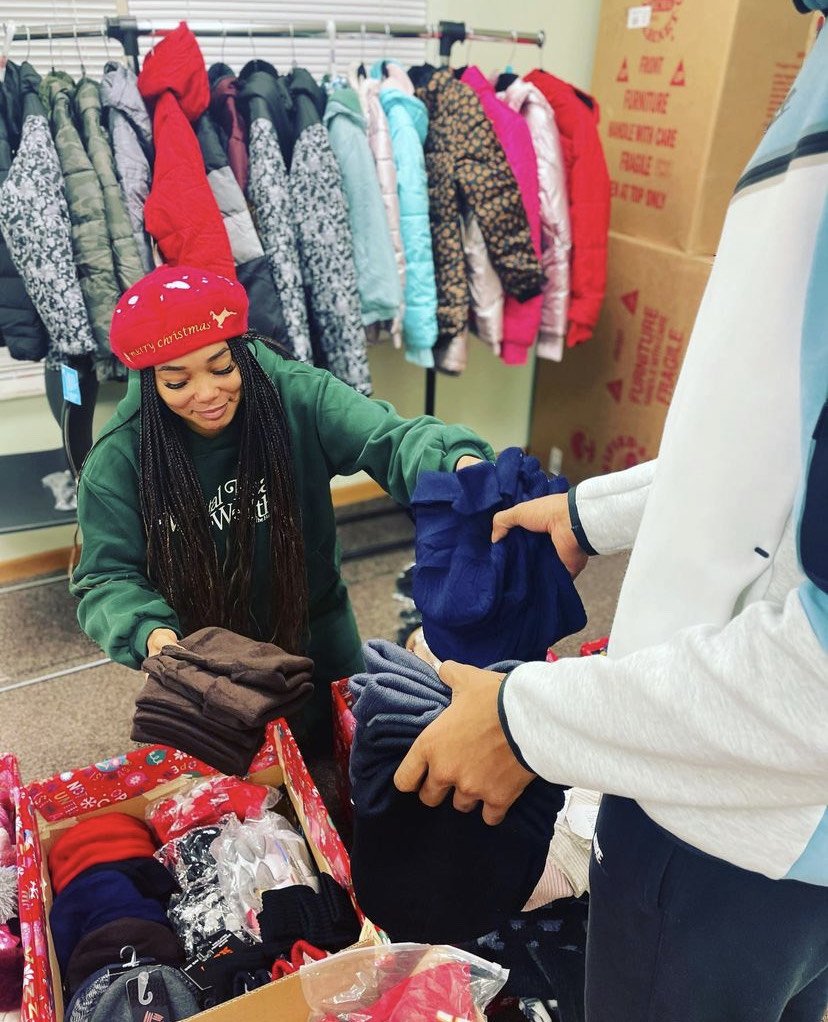This detailed photograph captures a bustling scene inside a donation warehouse or storeroom, likely around the Christmas season. Central to the image are two individuals handling various clothing items. On the right side, a man in a white sweatshirt is holding out a blue jacket and a gray wool garment, while his left hand grips another piece of clothing. Across from him, a woman wearing a red cap with "Merry Christmas" embroidered on it and a green sweatshirt is situated. She appears to be standing or crouching behind a table stacked with cardboard boxes adorned with festive Christmas decorations. Inside the boxes are wool hats and other winter accessories. In the background, a shelf brimming with multicolored winter coats on hangers—ranging from pinks and reds to blues and grays—adds depth to the scene. Large cardboard boxes labeled with care instructions, like "Handle with care" and "Fragile," are positioned to the right. The image's vertical orientation frames the well-organized chaos, highlighting the array of colors including red, green, blue, gray, and more, creating a vivid portrayal of a community effort to share warmth during the holiday season.